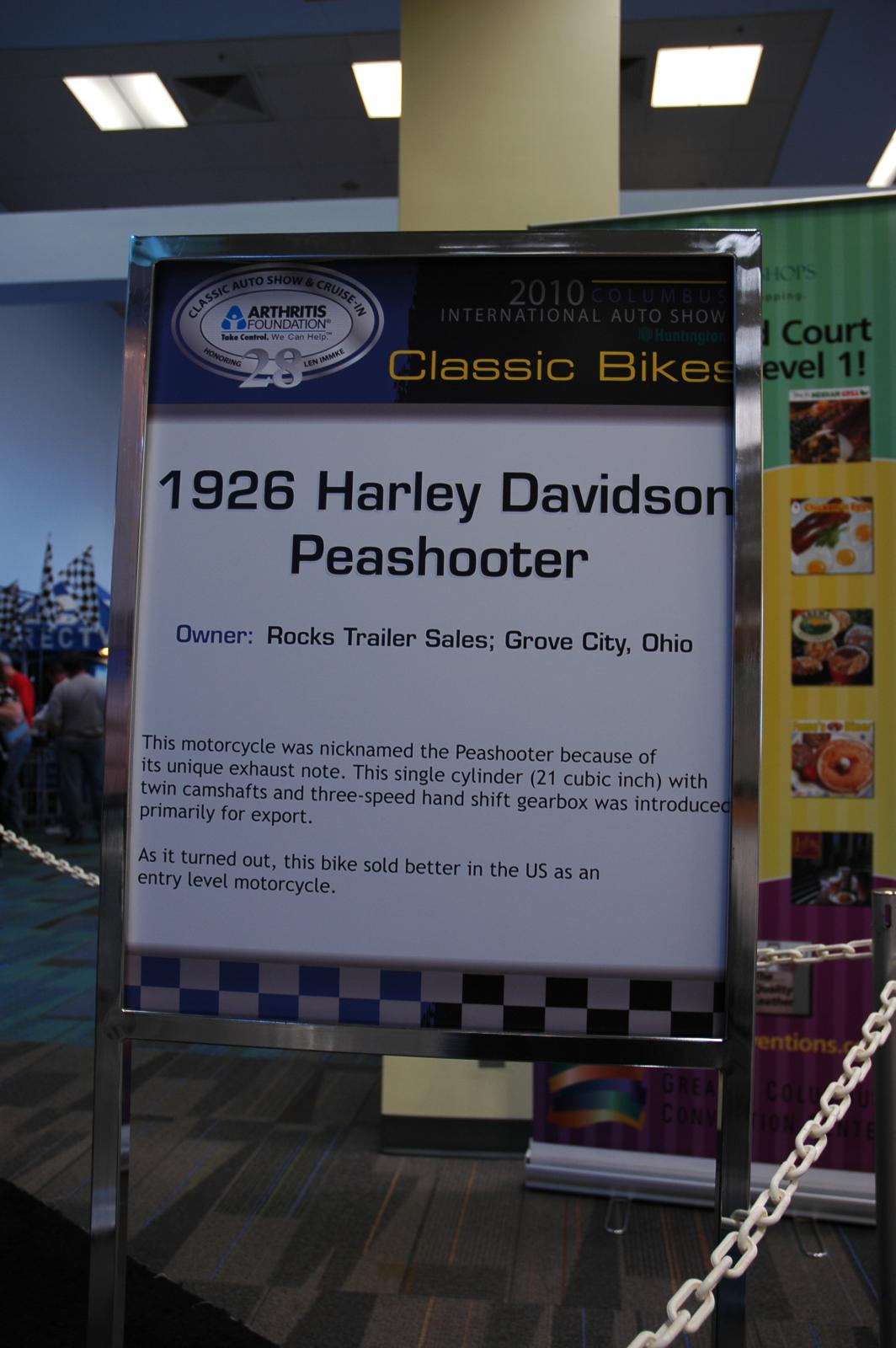The image features a detailed signboard located in what appears to be a busy convention or a food court with a false ceiling, lights, air conditioning vents, and a large pillar. Behind the sign, there's a banner showcasing various food items and text indicating "court level 11." The flooring beneath the sign is a design pattern common in malls or restaurants.

The sign itself is freestanding within a boundary set by small stands with chains and is held in a metal frame, standing approximately five feet off the ground. The top of the sign has a blue border, with "Classic Bikes" prominently displayed in yellow against a blue background. Above this, the year "2010" is written in white on a black background, and an oval logo in the upper left corner indicates the involvement of the "Arthritis Foundation."

The center of the sign provides key information about a "1926 Harley-Davidson Peashooter", owned by Rock Trailer Sales in Grove City, Ohio. The sign elaborates that this motorcycle was nicknamed the Peashooter due to its unique exhaust note and details its technical specifications, including a single-cylinder 21 cubic inch engine with twin camshafts and a three-speed hand shift gearbox. Originally introduced for export, the Peashooter found unexpected popularity as an entry-level motorcycle in the U.S.

This sign is part of a display that might be related to a classic bike exhibition, an auto show, or a sales event, given the detailed description and historical context provided. The presence of people standing or seated in the background, possibly looking towards a speaker or screen, and the adjacent pictorial signs hint at a dynamic, bustling environment.